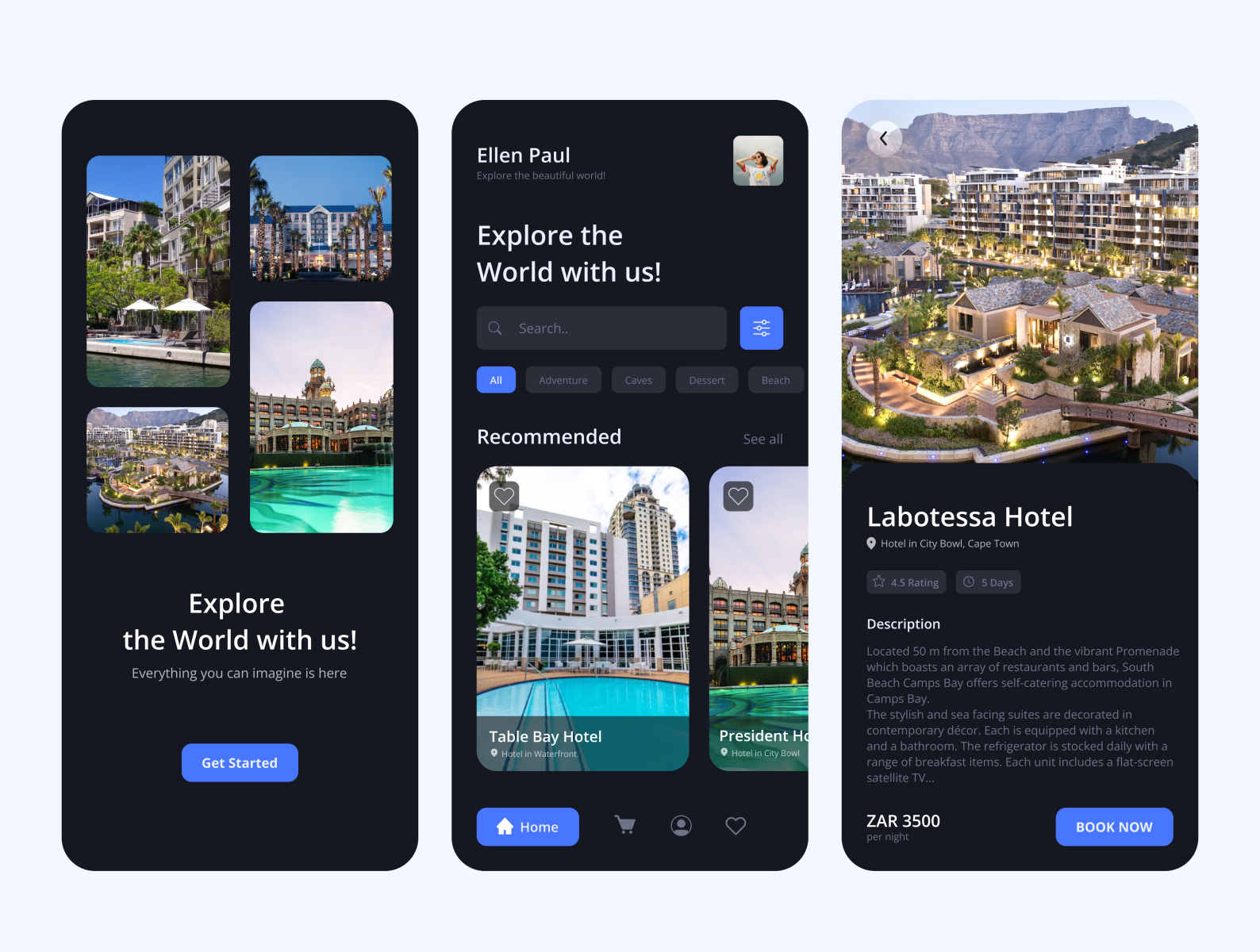The image displays three meticulously arranged screenshots against a black background, each presenting different facets of a travel-themed app or website.

On the left screenshot, there is a collage of four travel destination images, seamlessly separated by black space. The collage is structured with two images on top and two on the bottom; the left image in the top row is longer, and the right image shorter, with their lengths inversely mirrored in the bottom row. The vibrant photographs depict scenic vacation spots across foreign countries. Beneath the collage, there's white text stating, "Explore the world with us," followed by a smaller caption, "Everything you can imagine is here." Additionally, there's a prominent blue button labeled "Get Started" in white font.

The center screenshot features the profile of "Ellen Pohl" in white text on the left, accompanied by a small profile picture on the right. Below "Ellen Pohl," more white text repeats, "Explore the world with us." This section prominently includes a search bar, accompanied by a blue icon consisting of three lines and small circles, whose function remains unclear. Below the search bar, there are blue-highlighted filters labeled "All," "Adventure," "Caves," "Desert," and "Beach." The section titled "Recommended" showcases a picture of Table Bay Hotel and another somewhat indistinct image associated with a "President" caption, both adorned with a heart icon in the top-left corner. At the bottom, navigation buttons include a blue home button with a house icon, a shopping cart, a profile icon, and another heart icon.

The right screenshot highlights a picturesque nighttime scene of a lavish vacation destination, with illuminated buildings, water bodies, and surrounding mountains. The caption below reads "Lobotessa Hotel" in white text, with additional details noting a rating of 4.5 stars and a "3 days" reference, though further small text is unreadable. Underneath, two buttons and a brief two-paragraph description are visible, though too small to decipher. Finally, at the bottom, the text "ZAR 3500" is displayed alongside a blue button that states, "BOOK NOW" in white, capital letters.

This composition intricately weaves together a user-friendly interface, enticing travel imagery, and navigational elements designed to inspire and facilitate travel planning.